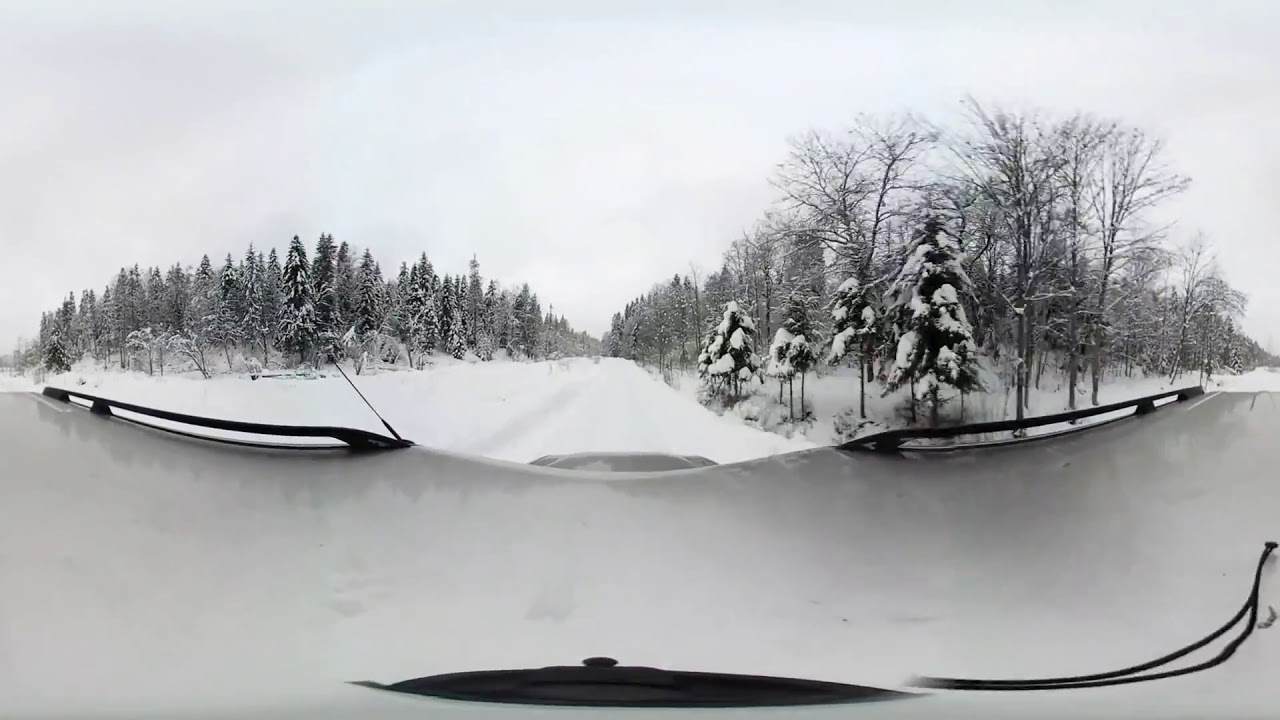This detailed black-and-white panoramic photograph captures a car driving down a deserted, snow-laden road. Taken from the windshield, the image showcases a mesmerizing winter landscape, with snow engulfing the unpaved road and creating a surreal 360-degree effect. The road curves to the right, revealing the snowy terrain behind the car due to the panoramic angle. Tall trees, their branches heavy with snow, line both sides of the road, resembling frosted Christmas trees, while leafless trees stand starkly against the sea of white. The car's headlights pierce through the snow-covered scene, its wipers frozen mid-swipe, emphasizing the harsh weather conditions. The sky merges seamlessly with the snowy ground, being equally white and overcast. There are no other cars or structures in sight, enhancing the sense of solitude and the captivating, almost ethereal beauty of this winter wonderland.